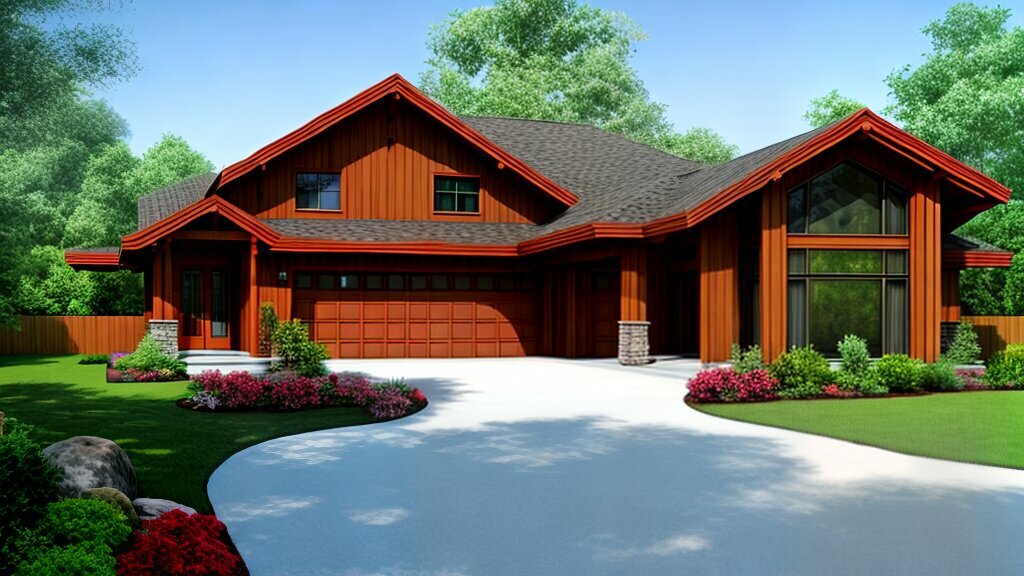This is a detailed depiction of a large, bright red wooden house with a distinctive architectural style that makes it hard to discern whether it's a photo or a painting. The house features a V-shaped gray roof lined with red shingles. On the left side of the house, there are double doors, and in the center, a large garage with two windows above it. The right side of the house showcases nearly floor-to-ceiling cathedral-style windows. The house is fronted by a long, bright white paved driveway that curves toward it, flanked by neatly manicured lawns and garden beds filled with green bushes and red and pink flowers. In the background, a wooden fence encloses the backyard, beyond which trees are visible, adding to the picturesque setting.